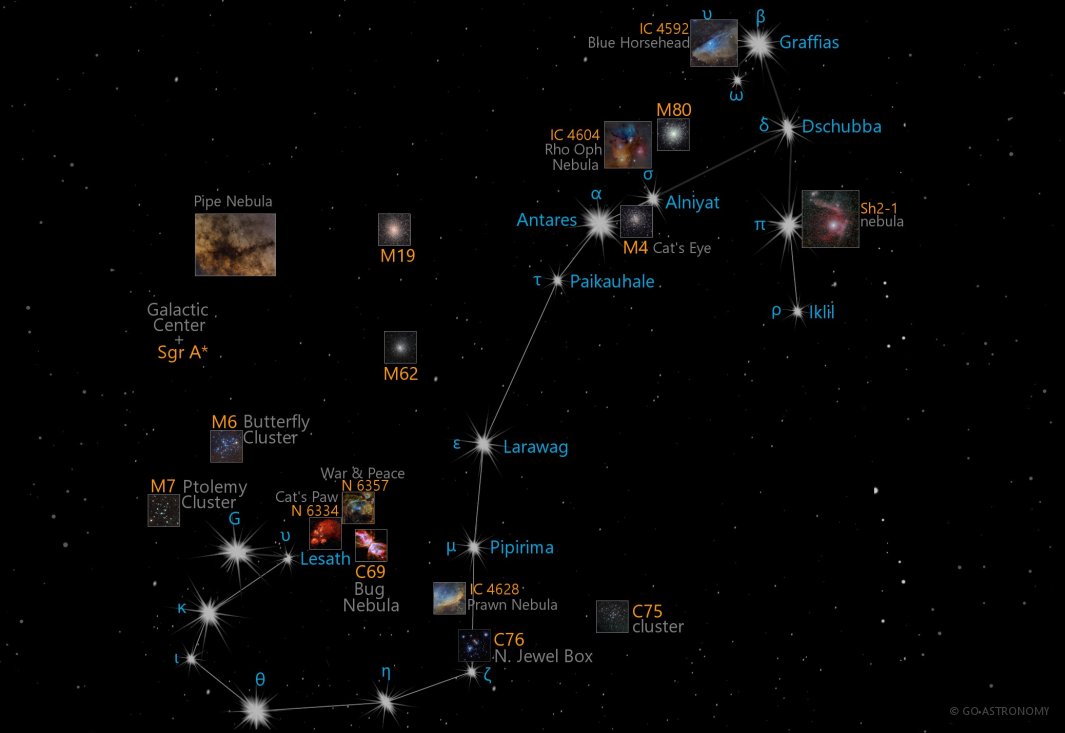The image showcases a detailed celestial map set against a black background with numerous tiny black dots. At the center, a white, zigzagging line weaves from the left to the bottom, then rises to the center right before descending again. This line connects various labeled white stars, creating a visually striking constellation chart. Notable stars include Lesath at the top left, along with U, K at the bottom, I, B, and KLILP towards the right center. The map also highlights significant celestial bodies and star clusters such as Larraweg, Pipurima, the Galactic Center, Bug Nebula, Butterfly Cluster, Antares, M80, C76 Jewelbox, C75 Cluster, Pipe Nebula, M19, and M62, all meticulously named against the dark sky canvas, enhancing the sense of navigating through the cosmos.